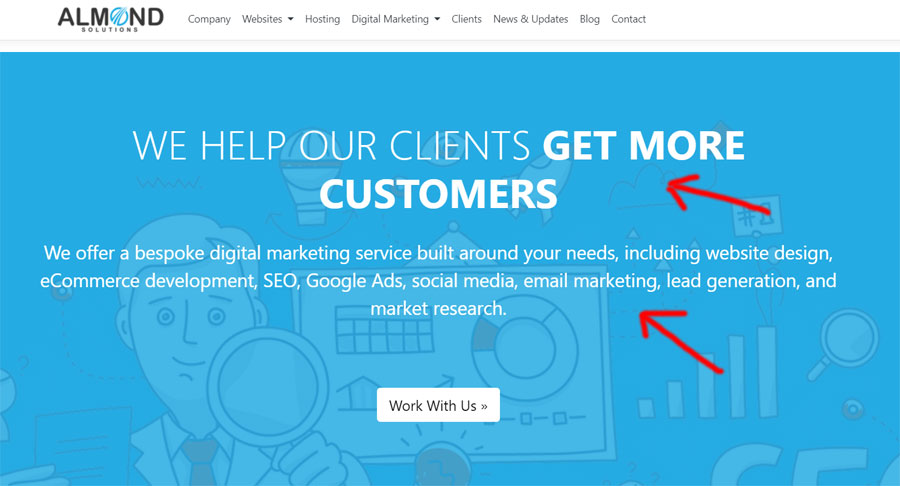Screenshot of Almond Solutions' Digital Marketing Services Webpage

The screenshot captures the homepage of Almond Solutions, a company specializing in digital marketing services. The top left corner prominently displays the Almond Solutions logo, accompanied by a navigation menu with links to various sections: Company, Websites, Hosting, Digital Marketing, Clients, News & Updates, Blog, and Contact.

Centered on the page is a bold, impactful headline that reads: "We help our clients get more customers," in large white font. Beneath this, a subheading elaborates on their offerings: "We offer a bespoke digital marketing service built around your needs, including website design, e-commerce development, SEO, Google Ads, social media, email marketing, lead generation, and market research."

A white call-to-action button labeled "Work with Us" is prominently displayed just below the subheading, encouraging potential clients to engage with the company.

The background of the webpage is light blue, adorned with subtle business-related illustrative graphics. These include a figure holding a magnifying glass, various charts, and red arrows that highlight critical points on the page. The overall design effectively communicates the company's comprehensive digital marketing solutions and creates a visually engaging experience for visitors.